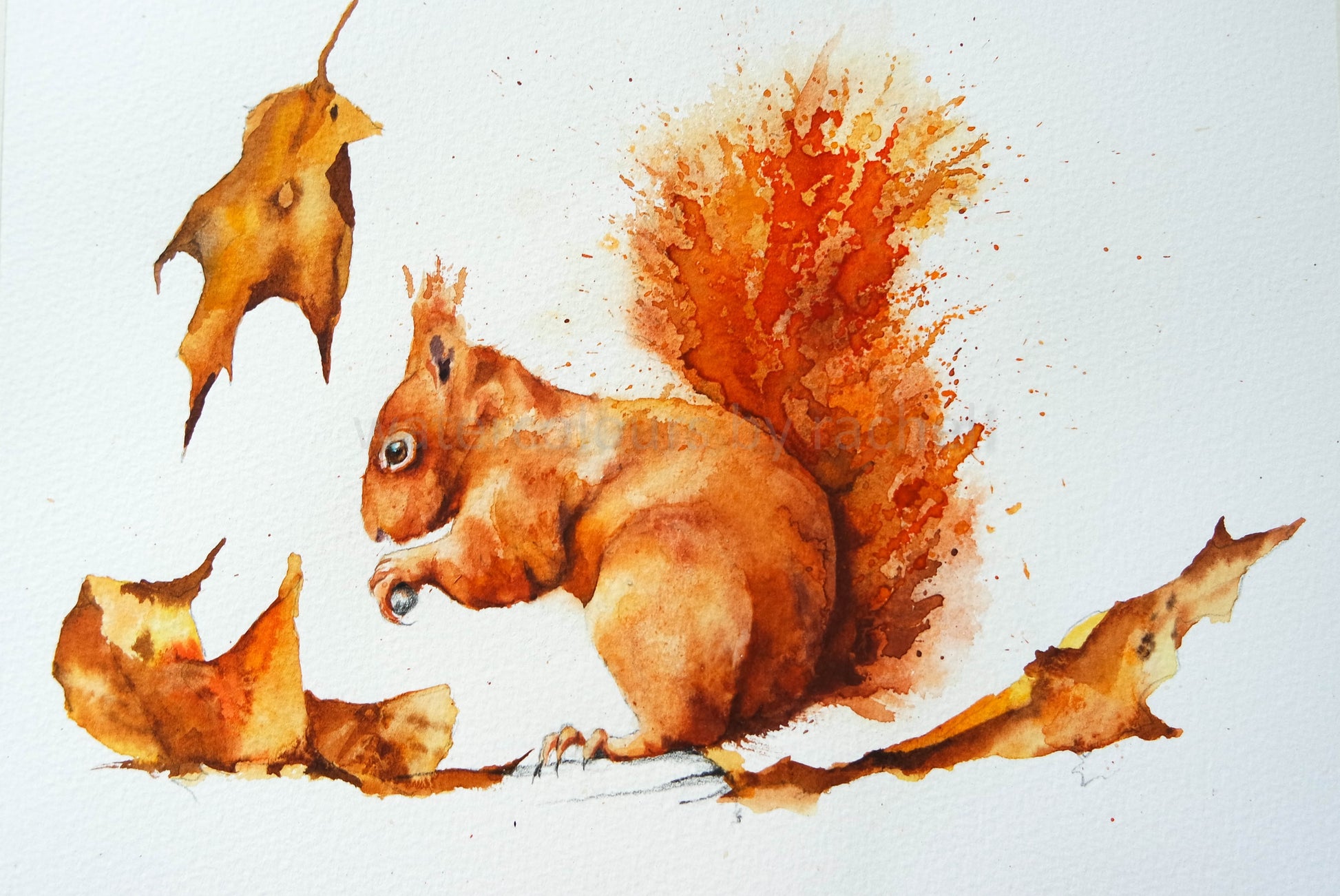The image depicts a watercolor painting featuring a finely detailed brown squirrel positioned centrally on an off-white canvas, with elements of canvas texture visible. The squirrel, oriented to the left, grasps a round, gray object in its paws while sitting upright. Its bushy tail is represented through an abstract blend of splattered brush strokes in vibrant hues of orange, yellow, and red, adding a dynamic element to the piece. Surrounding the squirrel, several leaves are rendered in varying states: one leaf, in shades of tan and brown, floats downward near the squirrel's head, while two other leaves, depicted with a more curled structure, rest on the ground in front of and to the right of the animal. A subtle splatter effect behind the squirrel's head enhances the overall whimsical and artistic style of the painting.